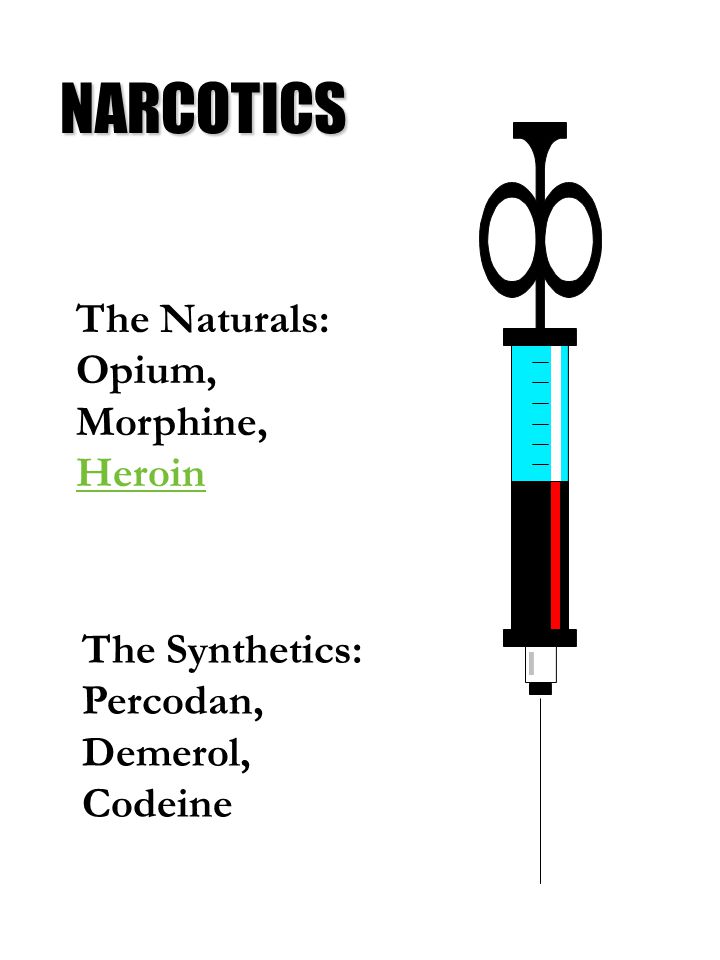This is an illustration of a hypodermic needle depicted on a white background. The needle, prominently positioned on the right side of the image and oriented downwards, features a black plunger at the top and a clear plastic barrel marked with black lines. Inside the syringe, there are varying colors, including black, blue, and a section filled with red liquid that resembles blood, while the needle itself is black and appears sharp and elongated. On the left side of the image, bold black uppercase letters spell out "NARCOTICS" at the top, followed by subheadings and lists in black letters: "NATURALS" listing "opium, morphine" and "heroin" in green letters, and "SYNTHETICS" listing "Percodan, Demerol, codeine". Overall, the image has a stylized, presentation-like quality with clearly delineated textual information contrasting the detailed needle illustration.